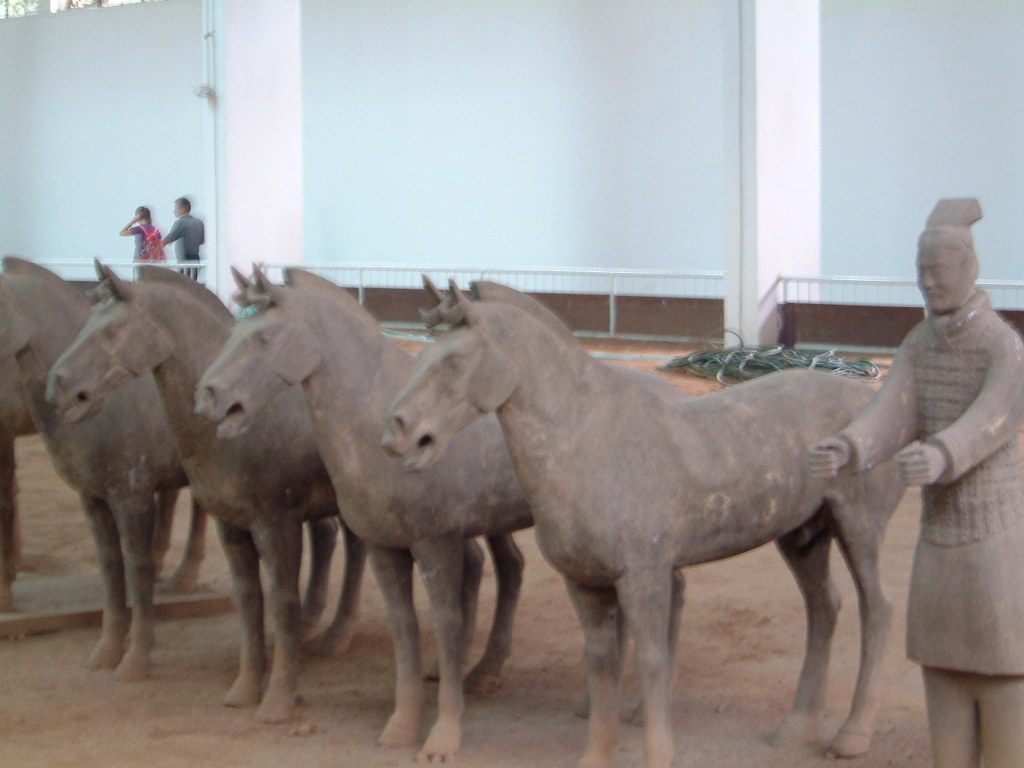In this photograph, we observe an impressive display resembling the famed Terracotta Army, prominently featuring five meticulously crafted life-size statues set on a reddish-brown surface. Positioned from left to right are four identical small horse statues, each standing upright on four legs, with their heads facing left and mouths ajar as if frozen mid-neigh. Standing to the rightmost side of the image is a statuesque figure of a man, dressed in what appears to be traditional Asian or Chinese attire, possibly a general, signified by his hat or hair styled into a rectangular shape extending from the back of his head. His stance is commanding with outstretched arms, though his feet are obscured. Both the horses and the man are constructed from dark terracotta, which mirrors the slight reddish tint of the ground they stand upon. The scene is set in a large, well-lit room with white walls and structural supports. In the distant left background, two people can be seen strolling behind a protective fence, which demarcates the display area from the viewers, adding scale and context to the grandeur of the statues.